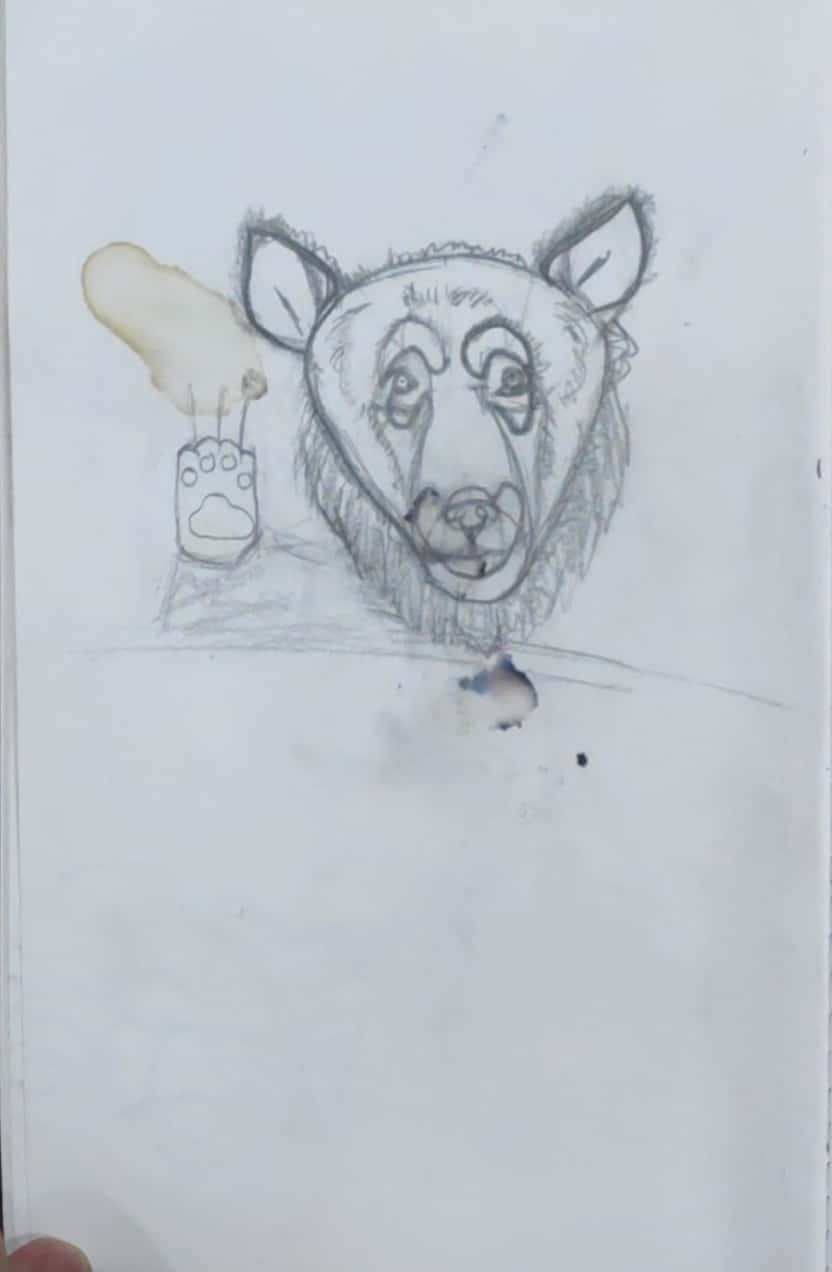A detailed pencil drawing of an animal, possibly a fox, dog, or lion, is depicted on a white piece of printer paper. The drawing showcases the animal's head and one of its paws, specifically the left paw from the viewer's perspective, complete with detailed claws. The illustration appears to be created with pencil. In the frame, a man's fingertip, likely his pointer finger, is visible holding the paper. The paper itself shows stains, including a small black circle, potentially made by paint, and a brown ring, possibly from a coffee spill or another beverage.